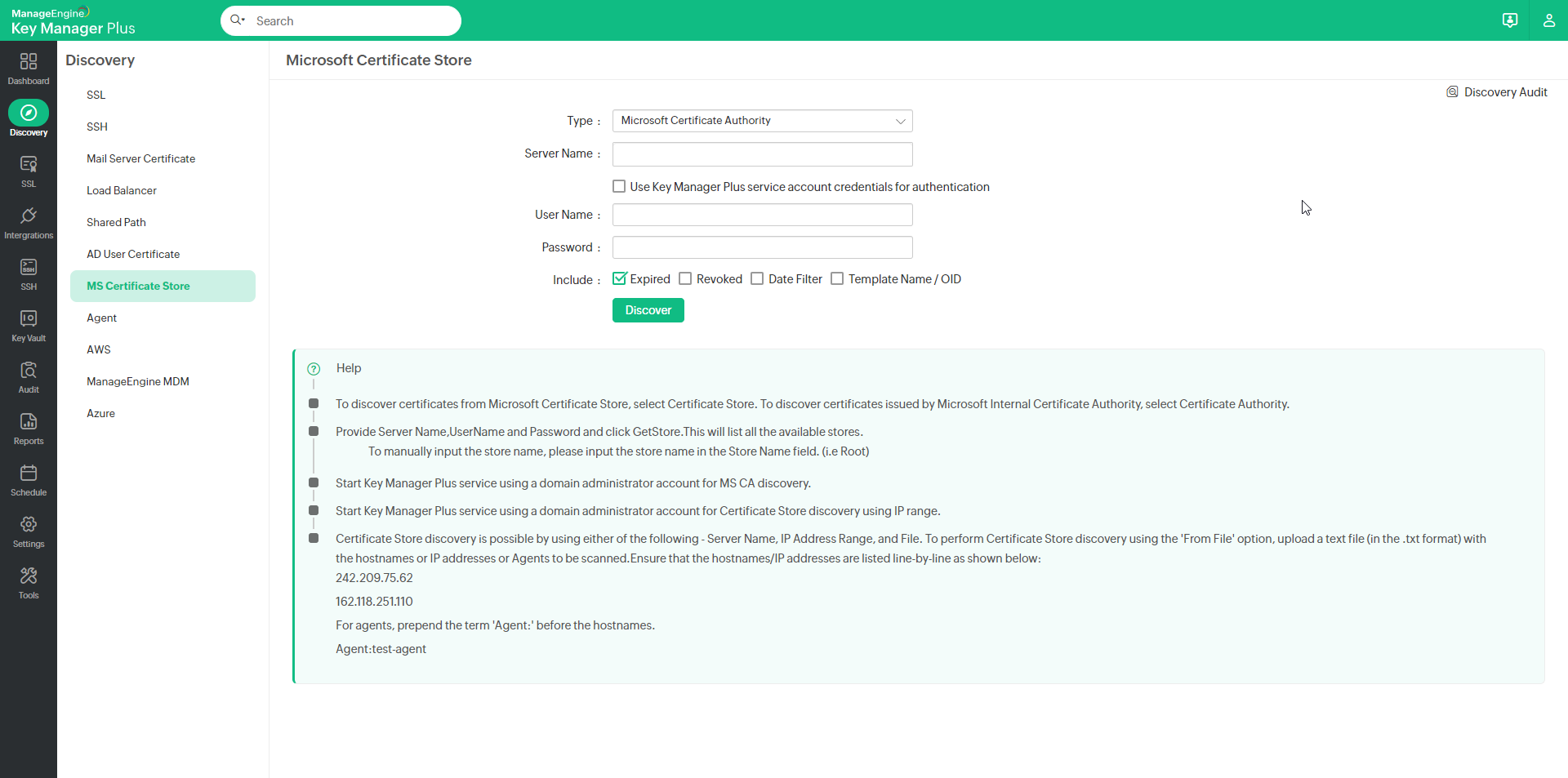The screenshot depicts a user interface within an online application, specifically "ManageEngine Key Manager Plus." The screen features a clear white background populated with various text buttons and interactive elements. The interface is divided into two main sections framed separately.

In the left frame, labeled with the title "ManageEngine Key Manager Plus" in black font at the top, there is a vertical banner displaying a series of menu icons. At the top of the banner, there is a house icon labeled "Dashboard." Below this, a round green icon precedes icons for "SSH," "SSL," "Key Store," and three additional unlabeled icons, each representing different functionalities or features within the application. 

On the right side of the image, the top portion displays a heading that reads "Microsoft Certificate Store." Directly beneath this heading, several dropdown fields are arranged vertically. These fields are labeled "Type," "Server Name," "User Name," "Password," and "Include," respectively. To the right of the "Include" field, specific options are displayed, detailing the parameters available for selection.

Overall, the image captures the detailed layout and organization of the ManageEngine Key Manager Plus interface, illustrating its user-friendly design and the various configurable options available for managing security certificates and keys.